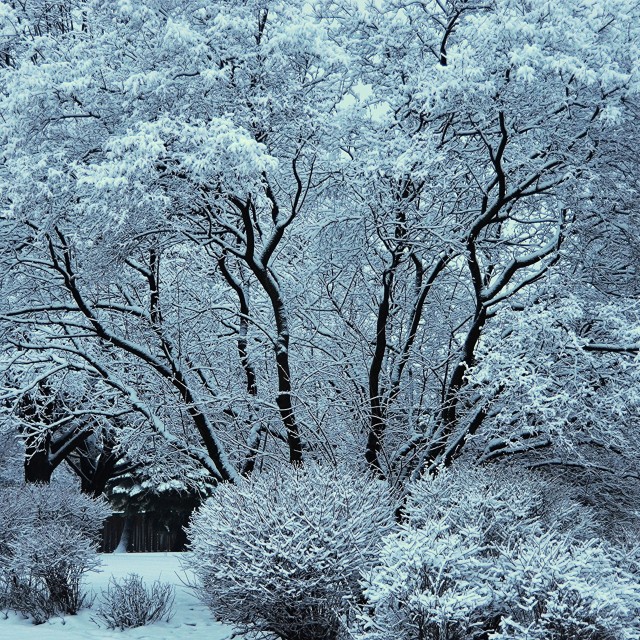The image captures a dense, snowy forest scene. The forest is thick with a variety of trees and shrubs, all heavily covered in snow. A prominent tree stands at the center, its dark brown or black branches spreading out in a wide V-shape and entirely cloaked in snow. Smaller bushes, also snow-drenched, dot the forest floor and create a slightly uneven landscape. The ground itself is blanketed in white, emphasizing the wintry setting. There is a small gap on the left side of the image, forming a slight pathway amid the snowy terrain. The overall palette is dominated by the white of the snow and the grey of the overcast sky, adding to the desolate, wintery atmosphere. The absence of any text ensures the viewer's focus remains solely on the serene and silent beauty of the snowy forest.